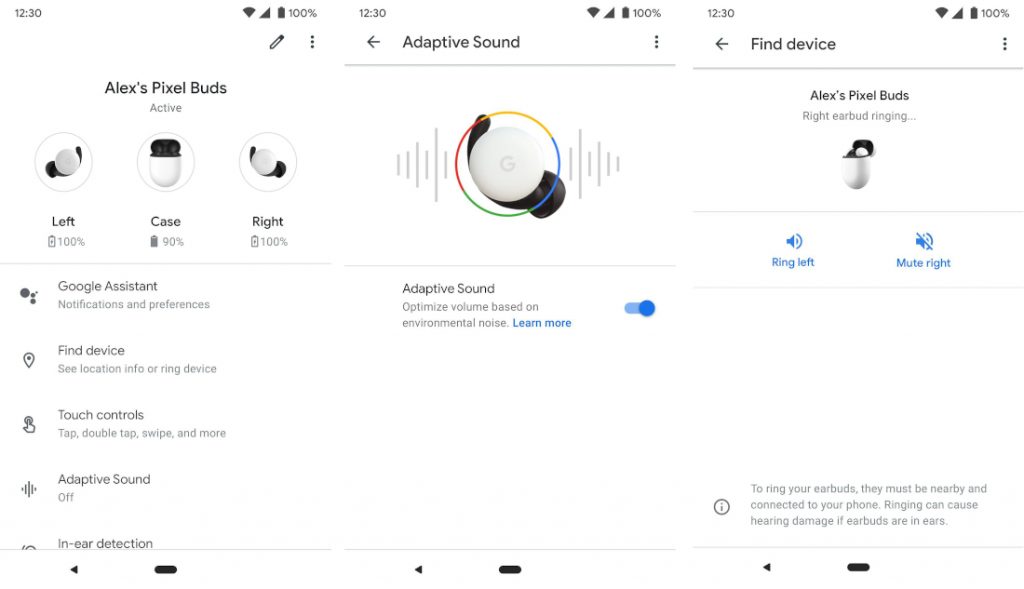### Detailed Caption for Image of Pixel Buds and Smartphone Screens

The image showcases three smartphone screen layouts, each uniquely displaying various settings and statuses related to Pixel Buds. All three screens feature phones with full Wi-Fi bars, full 4G bars, and 100% battery levels.

**Top Left Screen Layout:**
- The main title reads "Alexa's Pixel Buds Active."
- Subsections for battery information reveal that the left earbud and right earbud are at 100%, while the case is at 90%.
- Below these, several options are listed:
  - "Google Assistant" with settings for notifications and preferences.
  - "Find device" offers options to see the location info or ring the device.
  - "Touch controls" include functionalities like tap, double tap, swipe, and more.
  - "Adaptive Sound" is currently switched off.
  - "In-ear Detection" is positioned at the bottom.

**Middle Screen Layout:**
- This layout highlights adaptive sound settings at the top with a back button and a three-bar icon to the right.
- Centrally, there is an illustrative image of a Pixel Bud encircled by Google's iconic colors.
- To the right of the image, "Find device" is listed again, providing options for locating the Pixel Buds.
- It states "Alexa's Pixel Buds, right earbud ringing," with buttons below to "Ring left" and "Mute right," both in blue hyperlink text.

**Bottom Right Screen Layout:**
- Adaptive Sound settings are prominently displayed at the top.
- Below the image of the Pixel Bud is another adaptive sound status, showing it is enabled (checked).
- Sequentially, it follows with "Find device" settings.

Each screen layout provides a thorough overview of connected Pixel Buds' settings, emphasizing battery status, sound settings, device location, and control options.